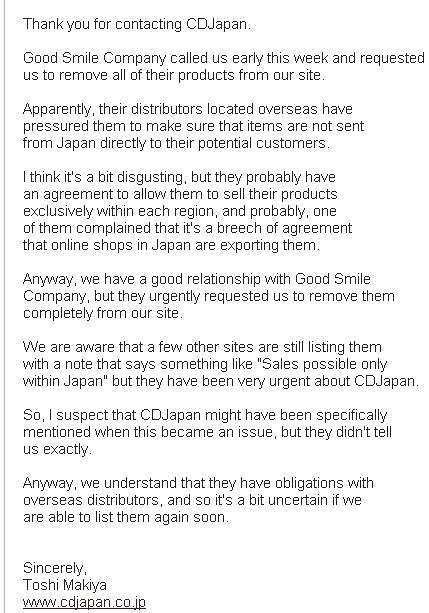The image displays an email from CD Japan, signed by Toshiya Makiya, addressing a customer's inquiry. The email explains that Good Smile Company contacted CD Japan earlier in the week to request the removal of all their products from the CD Japan website. This request stemmed from overseas distributors pressuring Good Smile Company to ensure that items are not sent directly from Japan to potential international customers. Although the CD Japan representative finds this situation unpleasant, they acknowledge that Good Smile Company likely has an agreement with regional distributors, which led to complaints of a breach when Japanese online stores exported products. The email notes that while other sites still list these products with restrictions like "sales possibly only within Japan," CD Japan has been specifically urged to comply. CD Japan values its relationship with Good Smile Company and understands their obligations with overseas distributors, though they are uncertain when or if they will be able to relist the products. The email also highlights a minor spelling error for the word "breach," which was incorrectly spelled as "breech."